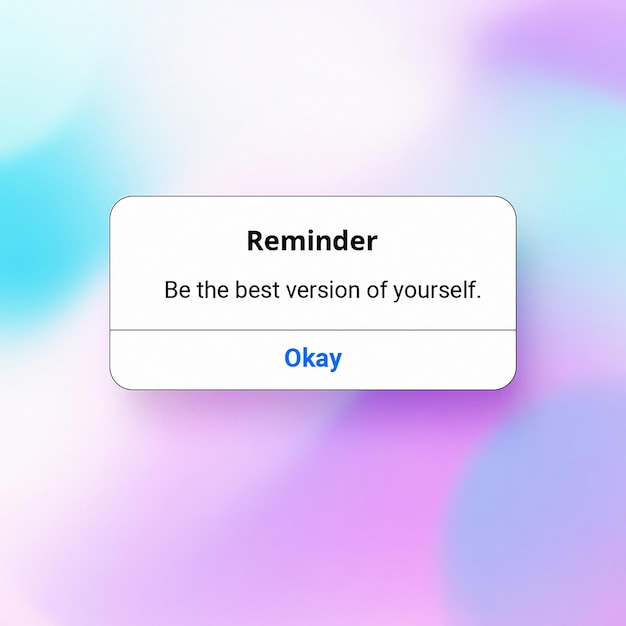The image features a background with a blend of turquoise, teal, white, light purple, and dark purple shades, reminiscent of the vibrant designs found on 90s cup patterns. The colors merge together in a manner that resembles a tie-dye effect. At the center, there is a white rectangular box with a sharp, black outline. Inside the box, "REMINDER" is written at the top in bold black text. Beneath it, in smaller, non-bold letters, appears the phrase "Be the best version of yourself." A horizontal line runs across the box underneath this text. Centered below the line, the word "OK" is displayed in blue font. The design is clean and focused, with no other elements present.